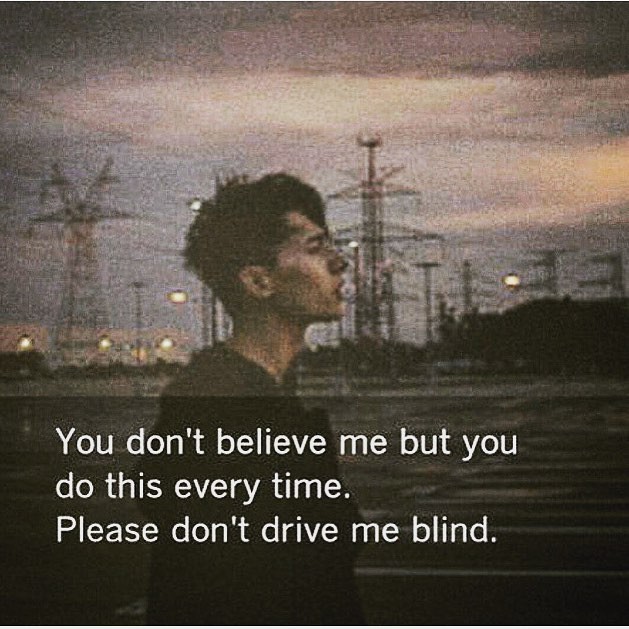In this artistic photograph, a young Caucasian man with short black hair, wearing a dark-colored shirt, is the central focus. His lips are pursed, and he's looking towards the right side of the image. The background features high voltage power lines with metal towers and scattered street lamps, running diagonally across a sky that appears dull and gray, indicating dusk or dawn. The bottom third of the image is slightly darkened, framing a poignant quote in white text that reads, "You don't believe me, but you do this every time. Please don't drive me blind." The overall image has a grainy and slightly blurry quality, adding to its moody and evocative atmosphere.